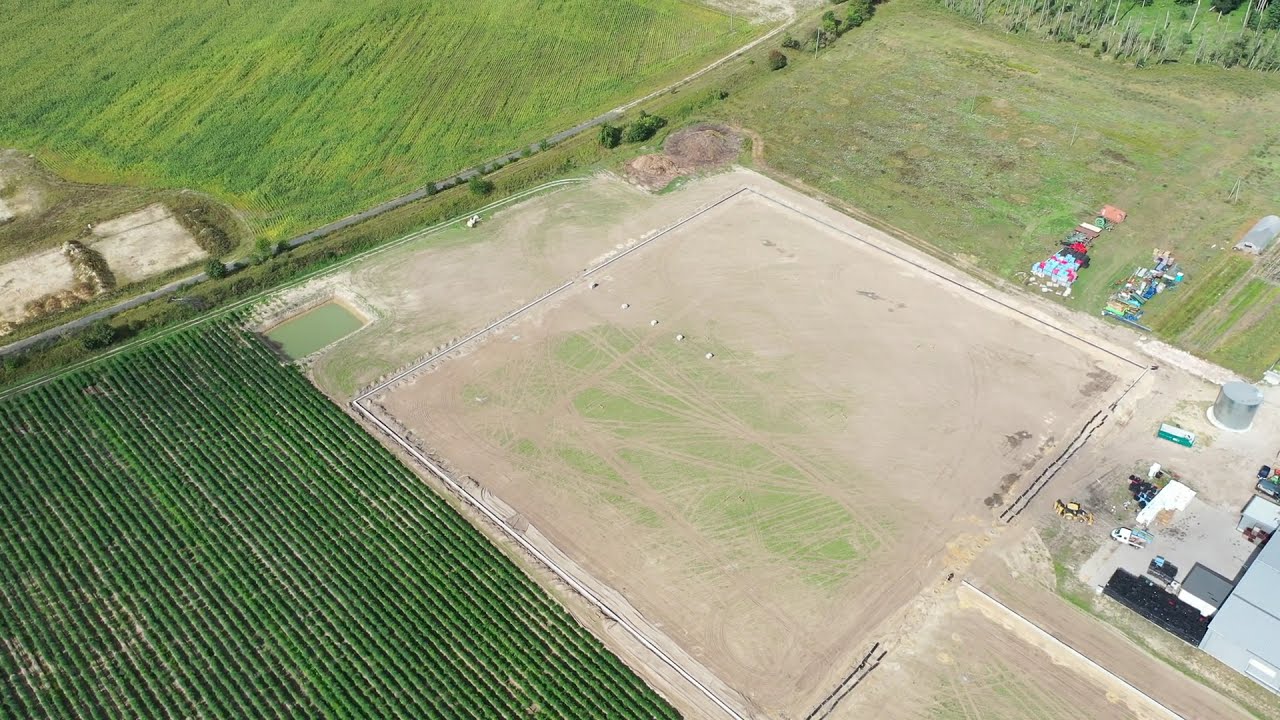The image captures an elevated view, approximately 50 feet off the ground, of a divided farmland. In the upper left corner, there is a lush green farm, while the left side of the image shows distinct rows of verdant crops. Dominating the center is a barren, square plot of land, which is enclosed by a network of pipes; the pipes along the bottom left, upper left, and upper right edges are white, while those on the upper right side appear black. At the bottom of this central plot, two white pipes veer slightly right before transitioning into black pipes. To the right of this central plot is a partial view of a gray building, fronted by a concrete slab. A white pickup truck is parked on the slab, and nearby, slightly above and to the right, a silver cylindrical container is visible. The bottom left corner of the image also shows a portion of another plot with green rows, adding contrast to the predominantly earthy tones.